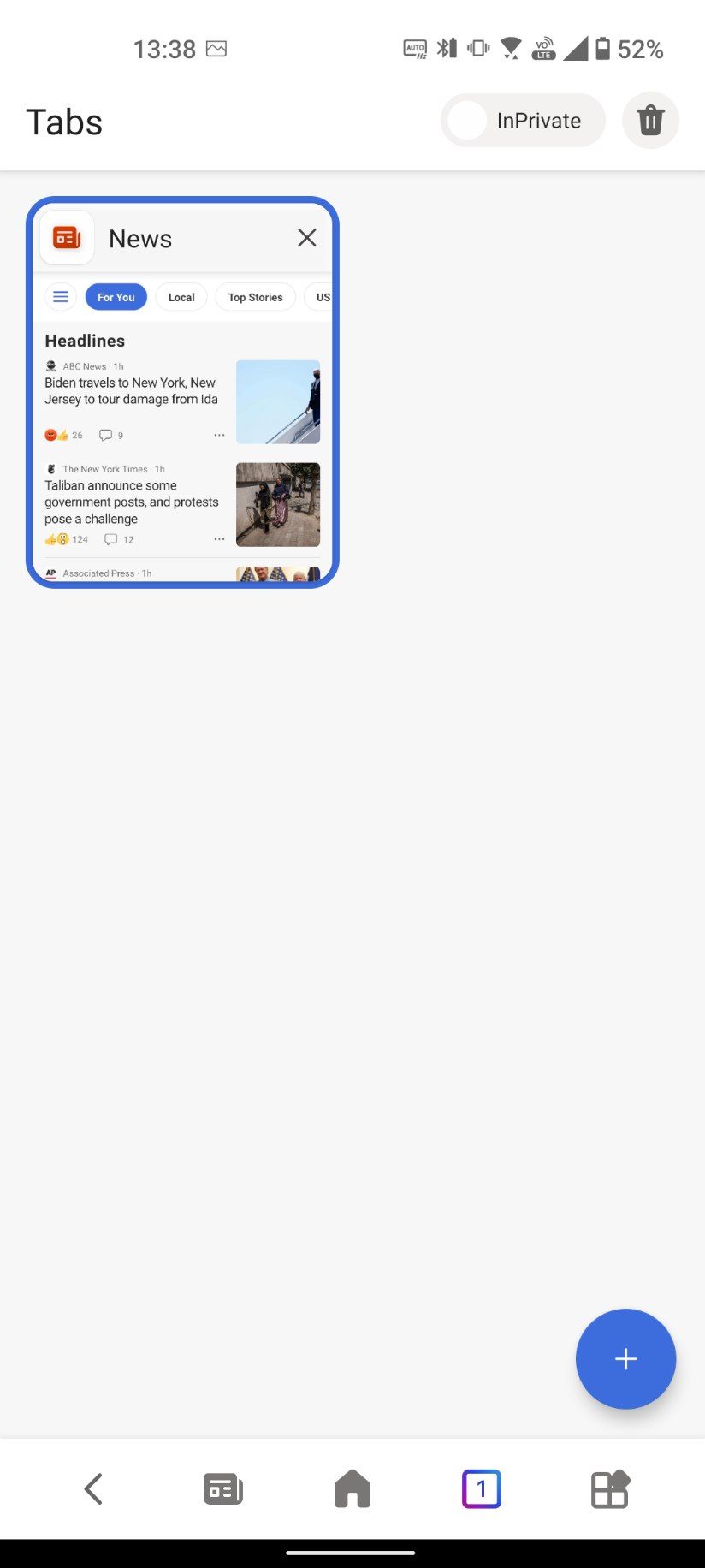The image showcases a phone screen with a predominantly white background. At the top, the screen displays standard icons in black, including the time, Wi-Fi signal strength, cellular signal bars, and battery level. Below these icons, the text "Tabs" appears in black, accompanied by a toggle button labeled for "InPrivate" browsing, and an icon resembling a trash bin.

In the upper left portion of the screen, there is a highlighted vertical rectangular section titled "News," marked in blue with an "X" closeout button to its right. This section contains news headlines, one concerning President Biden with an image of him descending the steps of Air Force One, and another about the Taliban, featuring indistinct images of two individuals.

The rest of the screen is white except for a blue circle with a white plus sign at the bottom, indicating the option to add a new tab. Additionally, a series of navigation icons is displayed at the bottom: a left-facing arrow for "Back," an icon resembling a newspaper for "News," a "Home" icon, a square with the number "1" inside it, and another square divided into four quadrants with one quadrant blacked out and tilted.

A thin black banner with a white line running through its center is displayed just above the navigation icons, suggesting the functionality to swipe up and return to the home screen.